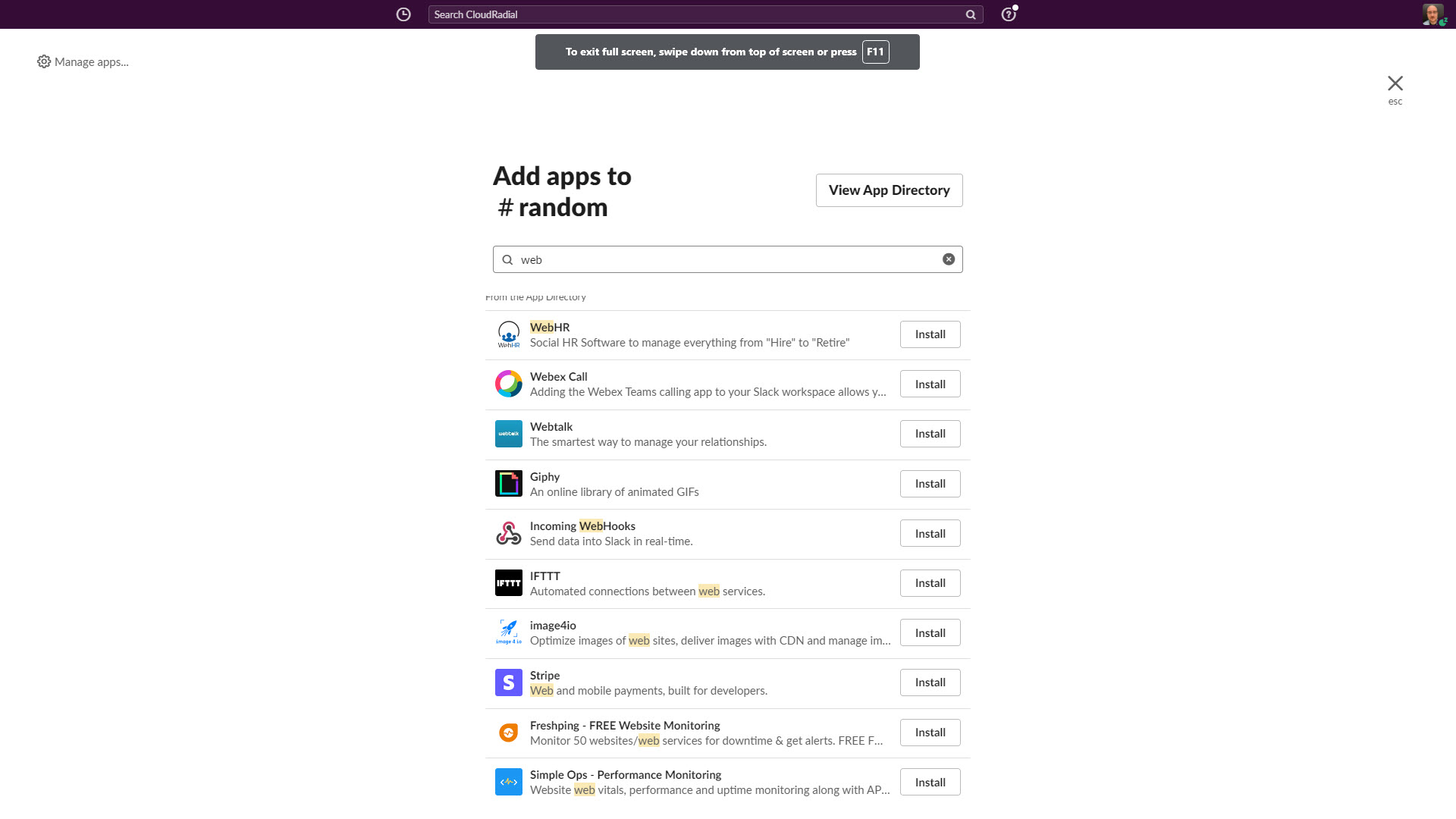**Detailed Caption:**

The image is a detailed desktop screenshot displaying a web interface, likely belonging to either a website or a system settings dashboard. At the top of the screen, a distinctive purple bar features various utility elements: a clock, a search field labeled "Search Cloud Radio," and a question mark icon with an accompanying notification alert. In the top left corner, a user profile image of a white, balding man indicates that a user is signed in. Adjacent to the profile icon is a cogwheel icon labeled "Manage Apps." 

An instruction banner stretches across the top of the screen, guiding users on how to exit full screen mode—by swiping down from the top of the screen or by pressing F11. Toward the upper right corner, there is an "X" icon, providing a shortcut for users to close the full screen view.

Beneath these elements, a heading prompts users to "Add Apps to #random view App Directory," supported by a prominently placed, white rectangular search box filled with black text. The user appears to have searched for apps related to the term "web," with several search results displayed sequentially. 

1. **WebHR**: Described as social HR software, it aims to manage every aspect from hiring to retirement.
2. **WebEx Call**: Offers the ability to integrate the WebEx Teams calling app into a Slack workspace.
3. **WebTalk**: Marketed as an effective tool for managing relationships.
4. **Giphy**: An online library of animated GIFs.
5. **Incoming Webhooks**: Sends data into Slack in real-time.
6. **IFTTT**: Facilitates automated connections between various web services.
7. **Image4IO**: Helps optimize website images, delivers them through a CDN, and manages them efficiently.
8. **Stripe**: Renowned for providing web and mobile payment solutions designed for developers.
9. **FreshPing**: Monitors up to 50 websites for downtime and provides real-time alerts.
10. **Simple Ops**: Offers performance monitoring for websites, covering web vitals, performance, and uptime.

The text indicates that these applications can be added either to the user's computer or as browser extensions, enhancing functionality and user experience.